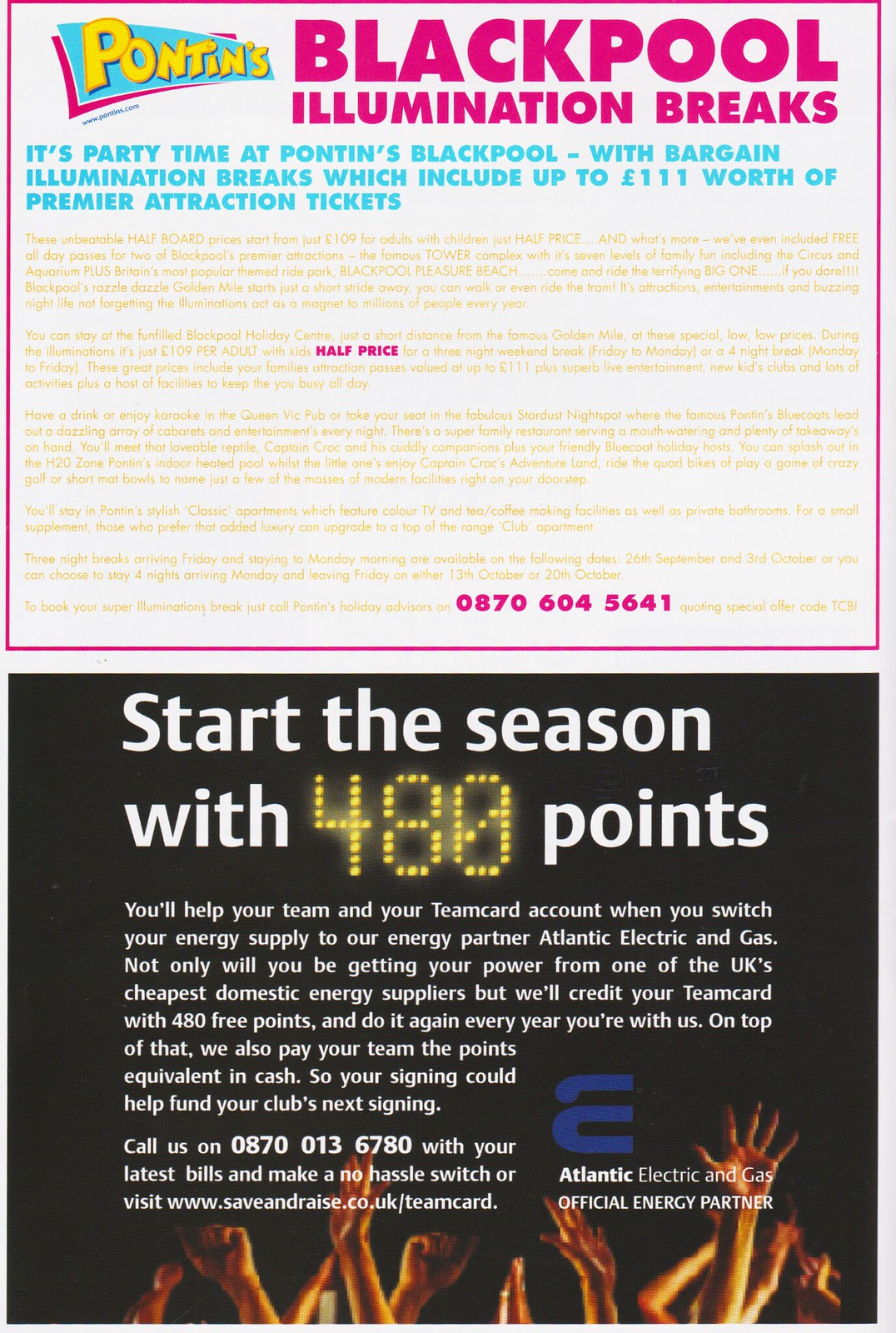The flyer is divided into two main sections, each serving different promotional purposes. The top section has a white background featuring the Pontins logo in yellow text with a blue flag. It announces "Pontins Blackpool Illumination Breaks" in dark pink/magenta letters. Below, it reads in blue, "It's party time at Pontins Blackpool with a bargain Illumination Break, which includes up to £111 worth of premier attraction tickets." There's additional small print in yellow that includes the phrase "half price" in bold magenta.

The bottom section has a black background with white text. At the top, it states "Start the season with 480 points," with "480" emphasized in yellow polka dots. This section relates to Atlantic Electric and Gas, the Official Energy Partner, and features an image of several arms raised in various gestures, including fists and jazz hands. The text at the bottom of this section provides instructions to "call us on 0870 013 6780 with your latest bills and make a no-hassle switch," and directs you to visit the saveandrace.co.uk team card for more information.